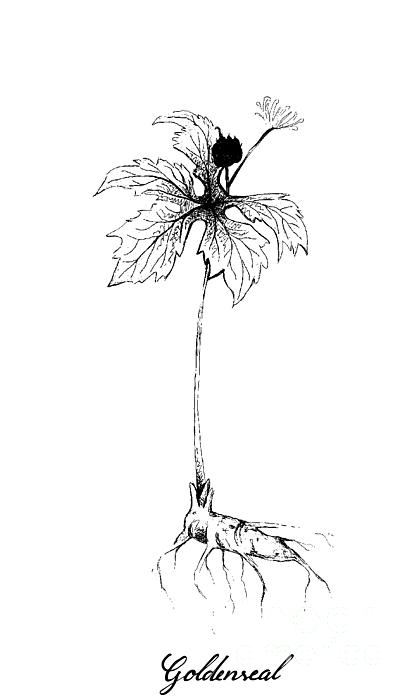The image is a detailed black ink drawing of a plant with a single stem, five leaves, and a central pistil, emerging from a thick, carrot-like root. The drawing is clear and monochromatic, placed against a white background with bright, even lighting. At the bottom of the image, in cursive black letters, is the word "goldenreal." The plant's stem extends upwards from the root, with one smaller stem bearing what appears to be a flower. The design is simple yet intricately focused on the root and flower elements, centrally positioned on the page.